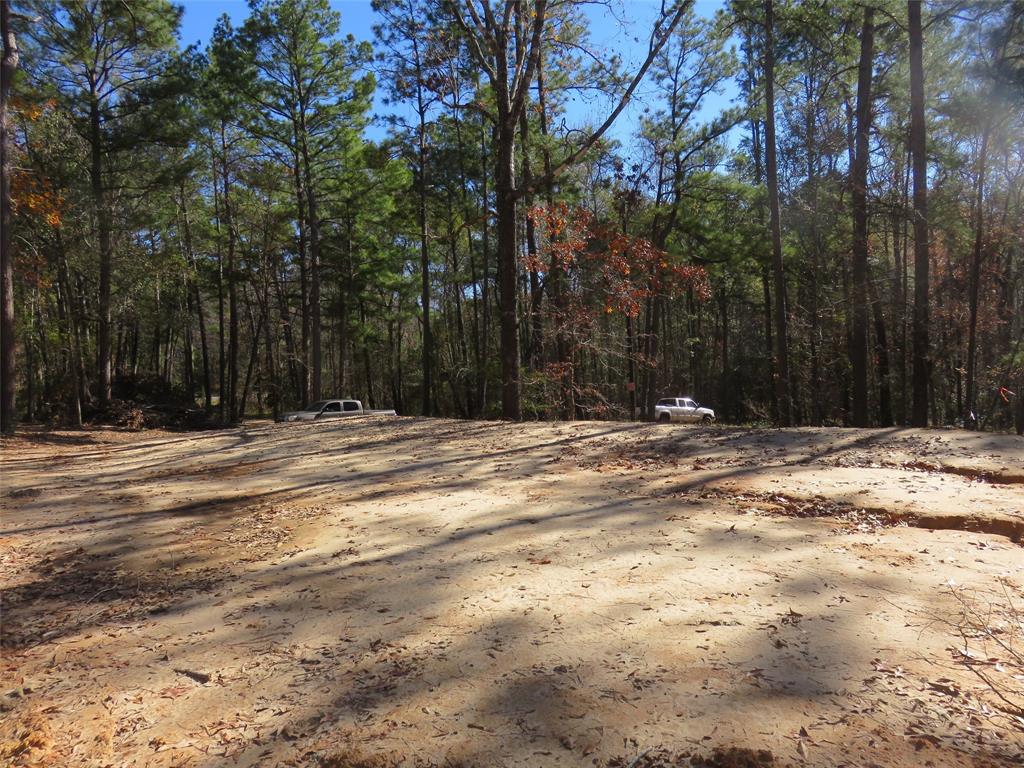In the bright outdoors, the image showcases a wide, open area covered in beige dirt scattered with dead leaves and twigs. This untouched plot of land occupies the forefront, suggesting it's a potential site for future construction. Dominating the background are tall pine trees with long, skinny brown trunks, interspersed with a few smaller trees bearing red leaves. The pristine blue sky peeks through the treetops without a cloud in sight. Two brown pickup trucks are positioned towards the middle left and middle right of the frame, facing opposite directions with their rears to each other, and reflections or shadows can be noticed. A slight haze on the right side adds a sense of depth to this harmonious natural setting.